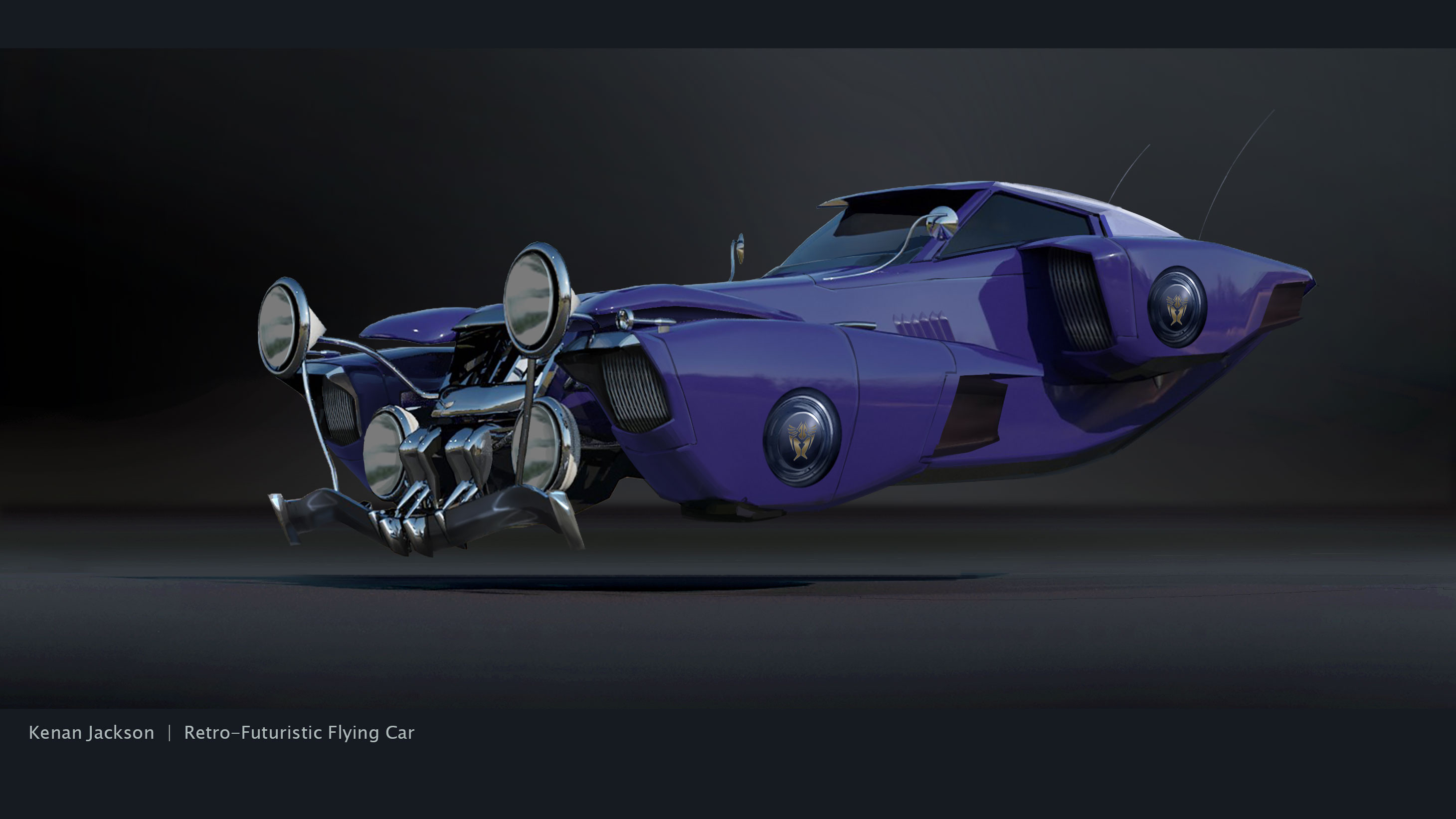This is a detailed digital rendering of a retro-futuristic flying car labeled "KENAN Jackson Retro Futuristic Flying Car." The image showcases a purple, two-door sports car floating approximately 16 inches off the ground against a gray, slightly darkened background that highlights the car's shadow. The vehicle resembles the body shape of a 70s Corvette with the front of an Oldsmobile and extensive chrome detailing, particularly on the grill and bumper. The front of the car features four round chrome headlights, two on each side of the tapered hood. Instead of wheels, the car has fenders that resemble wings, adding to its futuristic aesthetic. The sides are adorned with metallic, jet engine-like devices and two prominent silver circles. Accentuating its retro look, the car boasts a white convertible-style cloth top and two antennas protruding from the back. The rear appears to be lifted higher than the front, further emphasizing its ability to float.